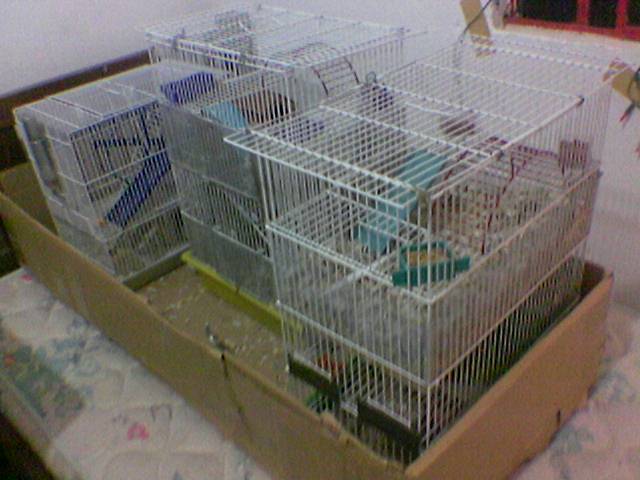The photograph captures three white animal cages, possibly for birds, arranged inside a cut-down cardboard box resting on a mattress against a wall. Each cage is outfitted with exercise wheels, blue ramps, and dual dishes for water and seeds, and they appear quite tall, narrow, and progressively shorter from left to right, with the middle cage being the tallest. A few scattered seeds are visible on the cardboard surface inside the box. A red-framed window is situated behind the setup, and there's a notable presence of debris inside the box, indicating the cages haven't been cleaned recently. The cages also feature miniature monkey bars, and one has a yellow plastic base. No animals are visibly present in the image.